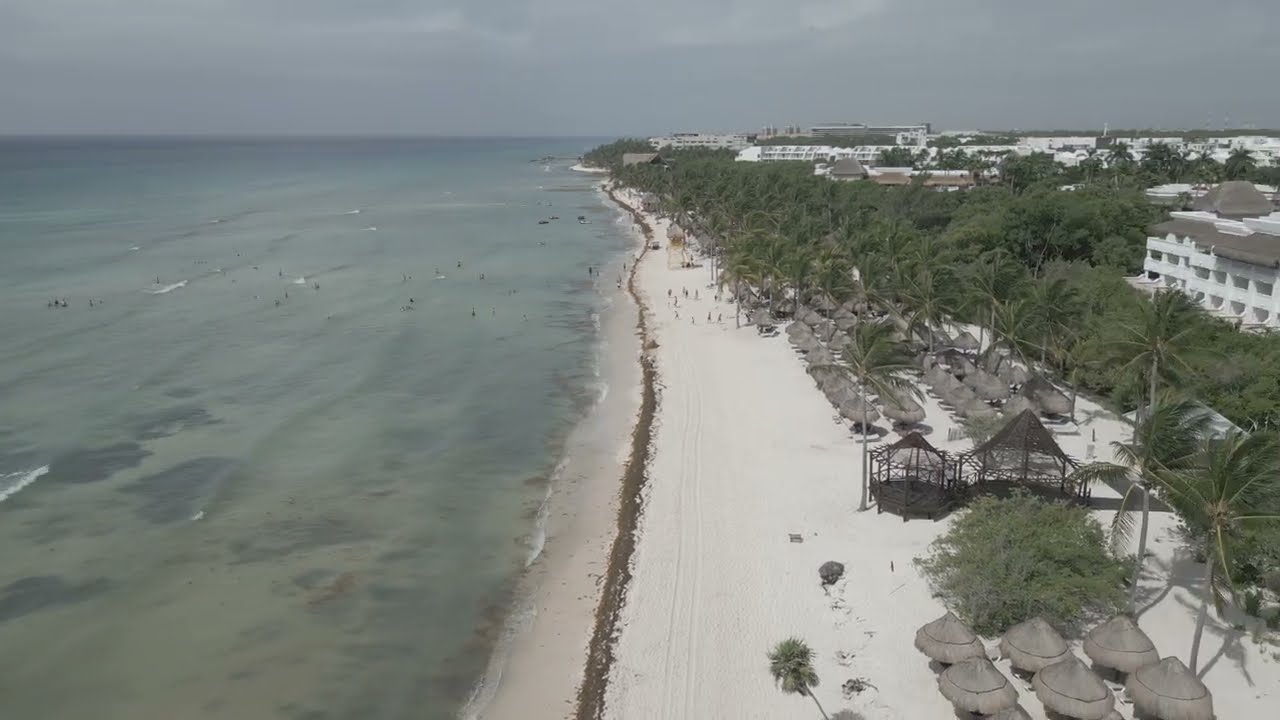The image presents an aerial view of a picturesque, tropical beachscape likely situated in a coastal city, possibly a popular tourist destination. On the left third of the image, a large, shallow ocean stretches across, its clear waters revealing subtle swells and a few small specks representing people swimming. The sandy beach occupies the central vertical strip of the picture, characterized by its pristine, white sand. Above the beach, the sky occupies the top eighth of the image, overcast with gray clouds.

To the right of the beach, several cabanas or huts are strategically placed, offering shade to beachgoers. These structures are scattered towards the bottom and middle sections of the image. Behind them, numerous tall, lush palm trees and other green foliage provide a tropical canopy. Further in the background, particularly towards the top right, a cluster of white buildings, likely resorts or hotels, rises, hinting at the area's allure for tourists. The entire scene exudes a tranquil, tropical charm, framed by the natural beauty of the ocean, the beach, and the lush greenery under a cloudy sky.